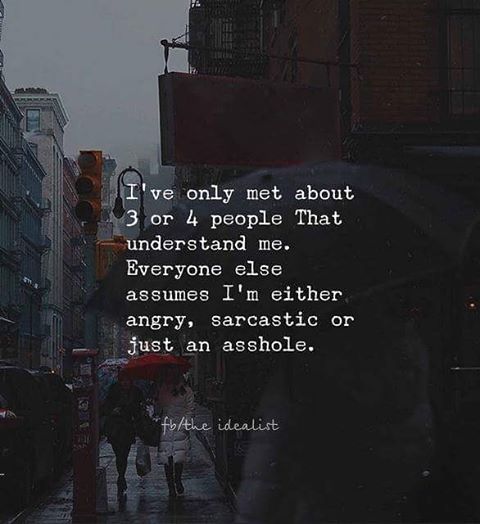The image captures a shaded, dark urban street scene with a rainy atmosphere. A dark vignette frames the image, which is populated by buildings to the left, including a distinctive black and tan building, a red brick building with either a fire escape or barred window, and cars parked along the street. Visible on the upper left is a yellow-housed stoplight. Prominently, there are people walking on the sidewalk. Two individuals are in focus, one wearing a white coat and carrying a red umbrella, and another in a black coat with a lighter-colored umbrella. A very out-of-focus umbrella possibly appears in the foreground, adding to the blurred, misty ambiance. A black pole with a sign featuring a white border and red center adds to the street’s urban feel. Inscribed in white text across the center of the image is a quote: "I've only met about three or four people that understand me. Everyone else assumes I'm either angry, sarcastic, or just an asshole," followed by "FB / The Idealist" at the bottom, suggesting a Facebook reference.